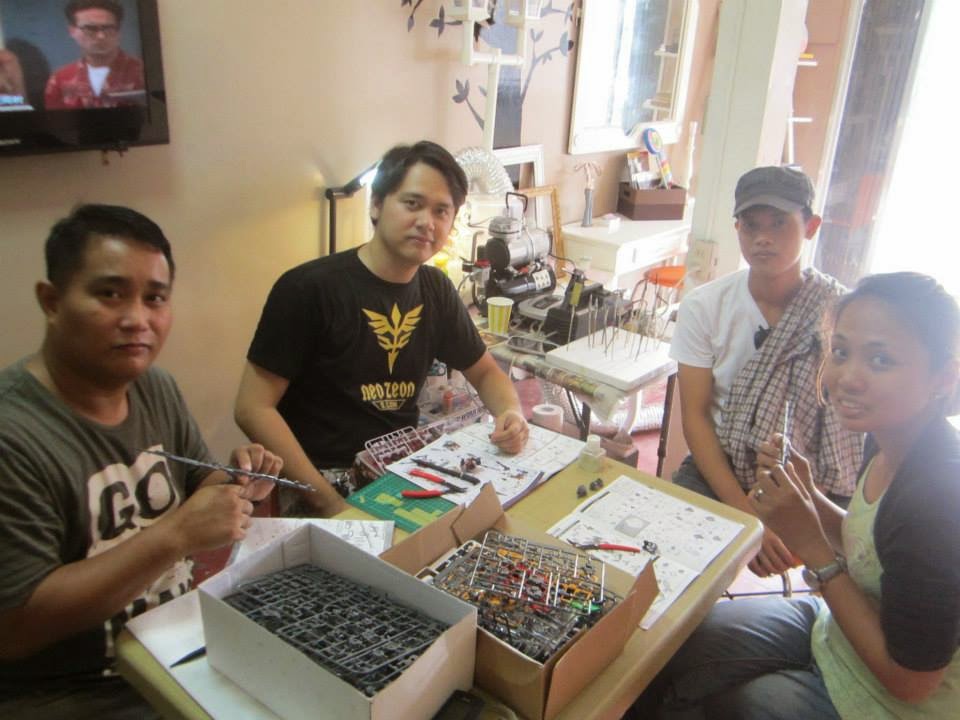In this detailed photograph, four individuals, likely of Asian descent, are gathered around a light tan table, engrossed in what appears to be the assembly of a model kit. The background features light peach-colored walls, with sunlight streaming through a window located in the upper right corner. The table is strewn with various colorful model parts, including gray, yellow, and red pieces, along with tools, small scissors, and instruction manuals. 

From left to right, we see the following people: a man with short black hair, wearing a gray shirt and looking directly at the camera; next to him is another man in a black t-shirt with a yellow "Neo-Zeon" decal, also facing the camera. Beside him, a man sporting a gray hat over a white t-shirt, layered with a plaid shirt, looks up from the table. The woman on the far right has dark brown hair, wears a black short-sleeve jacket over a light green shirt, and has an instruction manual in front of her.

The photograph includes several additional details: a corner of a TV is visible in the top left, while the top right reveals what seems to be a large door or window. In the background, a smaller table appears cluttered with various items, including sticks and a motor, hinting at the room's dynamic and industrious atmosphere.